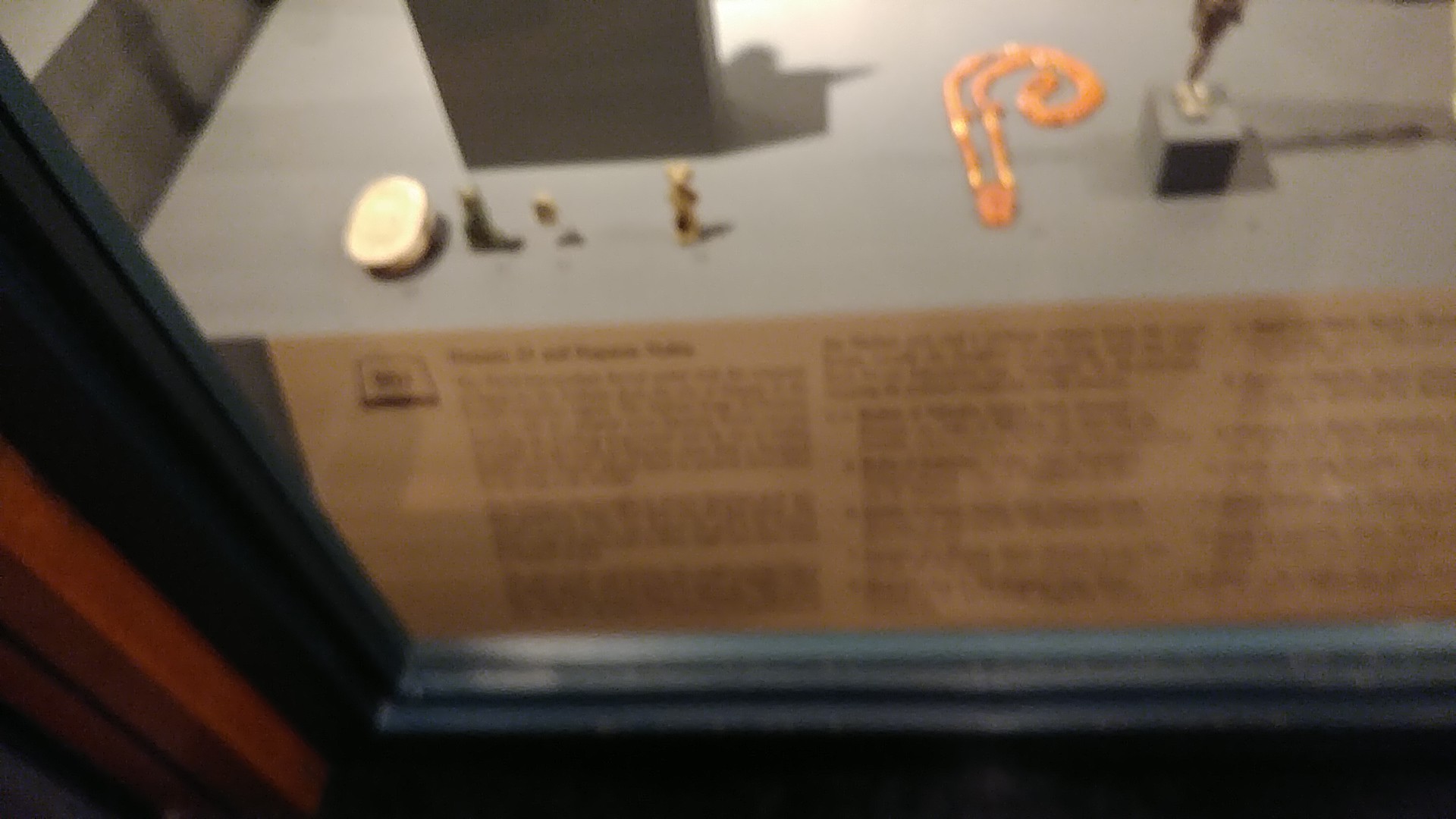The image features a room viewed through a blurry, possibly low-quality photograph that appears to be taken through a window or a two-way mirror, suggesting it might be an interview room or an exhibit space within a museum. Inside the room, a grey table holds an array of small items: a gold trophy casting a shadow to its right, a set of orange rosary beads without a cross, a black square box, and a few figurines. Pinned to the glass of the window or two-way mirror is a strip of paper with text that is illegible due to the blur. The overall scene gives an impression of displayed artifacts, each potentially holding a story obscured by the image's poor quality.